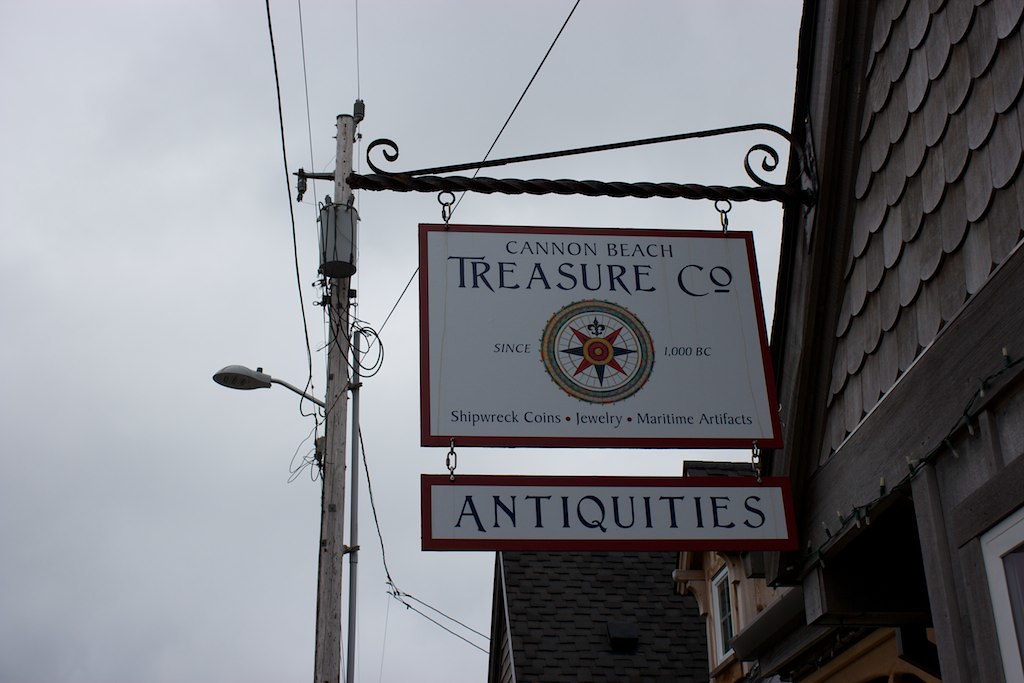The picture depicts a sign for the "Cannon Beach Treasure Company," hanging from a horizontal rod protruding from the roof of a storefront styled like a house with grayish-black wooden shingles on an A-frame roof. The main sign is rectangular with a white background and features the words "Cannon Beach Treasure Company" at the top. Below, there's a circular logo bordered in green and yellow, containing a multicolored star, flanked by the words "Since" on the left and "1000 BC" on the right. Beneath the logo, small text reads "Shipwreck Coins, Jewelry, Maritime Artifacts." Attached below this main sign by chains is a smaller sign stating "Antiquities." To the left of the building, there's a utility pole with a mounted light and web-like utility wires extending into a light gray sky. The overall image is in color, featuring a mix of red, white, gray, brown, and possibly blue or black hues, and is taken outdoors during daylight.